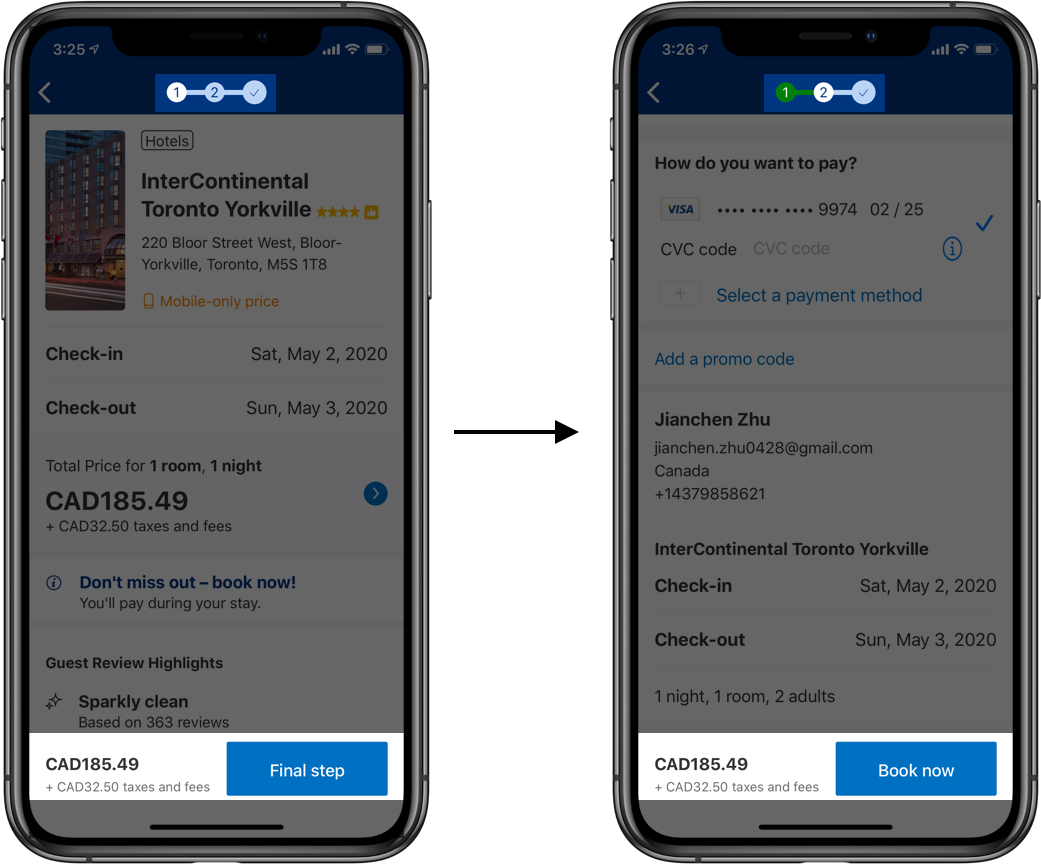The square image frame showcases two side-by-side screenshots of cell phone displays. Each phone is identifiable by its distinct frame, clearly visible within the image. Positioned between the two phones, a black arrow points from the left phone to the right, suggesting a transition or comparison.

Both phone screens have their main content grayed out, with a highlighted white pop-up banner at the bottom. In the left phone's display, the banner details the cost breakdown: "CAD 185.49 plus CAD 32.50 taxes and fees." To the right of this text is a blue button with white text that reads "Final Step."

The right phone's screen mirrors the cost breakdown: "CAD 185.49 plus CAD 32.50 taxes and fees." However, the blue button at the bottom says "Book Now." The grayed-out area surrounding the banner indicates that the user is viewing booking information for the Intercontinental Toronto Yorkville hotel, with check-in on May 2, 2020, and check-out on May 3, 2020.